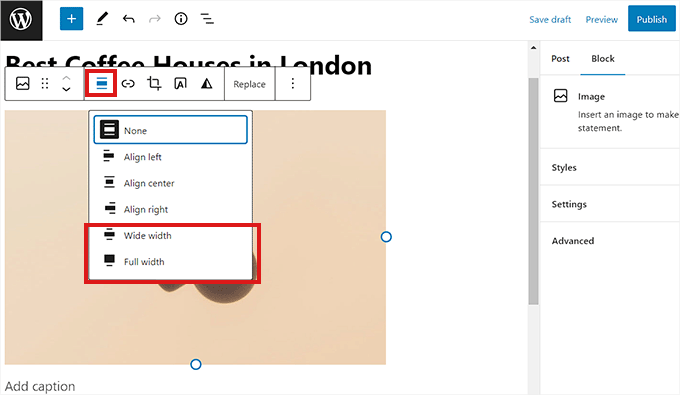In the upper left corner of the image, there is a black box featuring a white, capital "W" centered within a white circular outline. To the immediate right of this, a smaller blue box contains a plus symbol. Continuing rightward, there is a black pencil icon followed by left and right pointing arrows. Next to these arrows is a small circle with a lowercase "i" inside it, adjacent to three tiny diagonal lines.

Beneath these icons, partially obscured by an overlaying box, there is text which appears to read either "Rock Coffee House in London" or "Best Coffee House in London." The obstructing box has a visible red-outlined square section, alongside options to share, replace, and view additional options indicated by three vertical dots aligned in a column.

Down below, the word "None" is highlighted within a blue box. Further options beneath this text include "Align Left," "Align Center," "Align Right," and within a red outline, "Wide Width" and "Full Width." At the bottom left, there is text prompting "Add Caption." In the upper right corner, the word "Publish" is prominently displayed within a blue box.